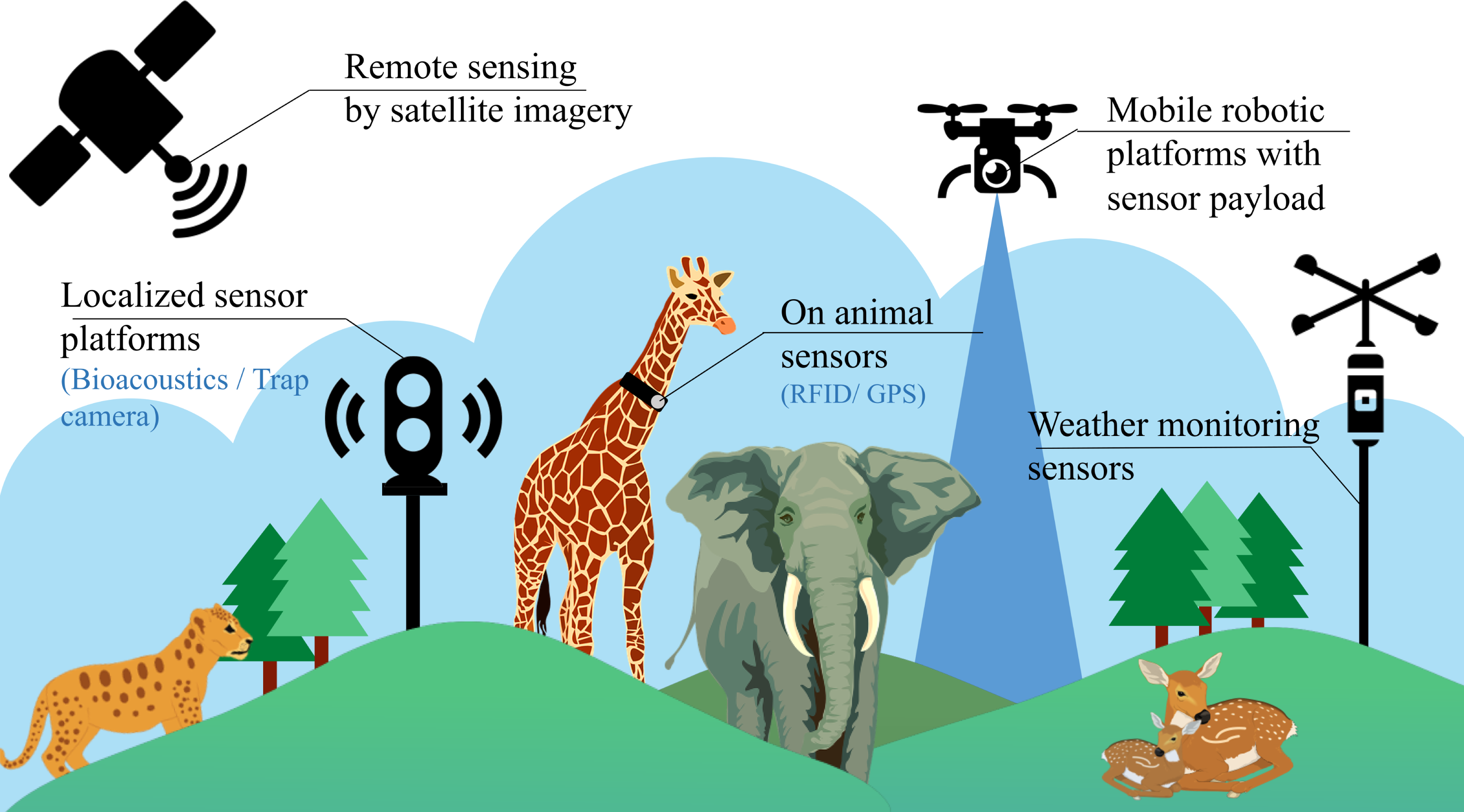The detailed illustration appears to resemble a textbook chart and features various zoo-like animals in a landscape with blue, mountain-like backgrounds. Prominent in the scene are a giraffe wearing a collar labeled “On Animal Sensors (RFID/GPS)” positioned centrally, and an elephant slightly to its right. To the left of the giraffe is a big cat, possibly a cougar. In the bottom right, a deer with its fawn is depicted. Overhead, a drone labeled “Remote Sensing by Satellite Imagery” hovers, while another drone-like device, resembling a toy airplane, is labeled “Mobile Robotic Platforms with Sensor Payload” situated above the elephant and slightly to the right. A black, stoplight-like structure between the cougar and giraffe reads “Localized Sensor Platforms (Bioacoustics/Track Camera).” Trees dot the landscape, and the colors throughout the image include green, blue, orange, black, white, and additional green and orange elements. Above the scene on the right, a tall structure with an "X" at the top is labeled "Weather Monitoring Sensors."